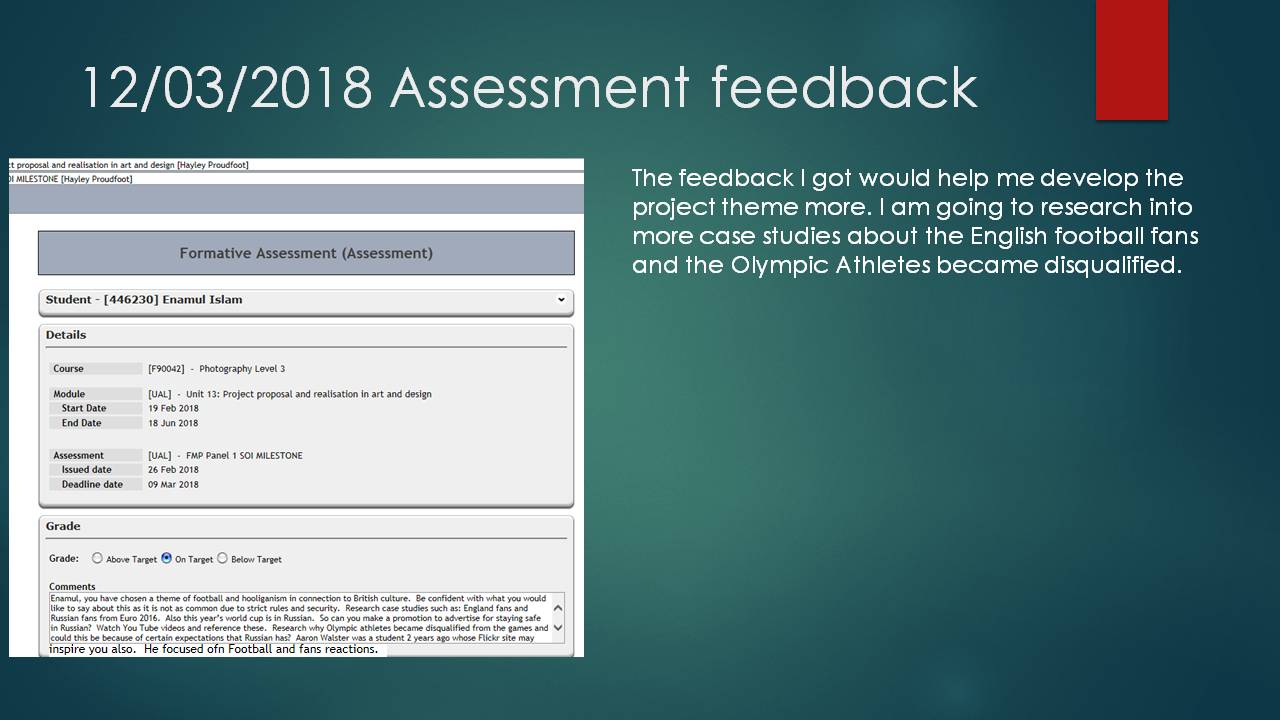The image is a wide rectangular PowerPoint slide with a greenish-blue gradient background, darker at the edges and lighter towards the center. Positioned in the upper left corner, the slide displays the date "12/03/2018" and the phrase "assessment feedback" in white font. A small red rectangle, resembling a bookmark, protrudes from the top right corner of the slide. Below the date and heading, on the left side, there is a square screenshot of a gray computer screen showing what appears to be a form or document, though the specific content is not legible due to its small size. To the right of the screenshot, in white font, the text reads: "The feedback I got would help me develop the project theme more. I am going to research into more case studies about the English football fans and the Olympic athletes became disqualified." The overall setup suggests that this slide is a part of a presentation, possibly detailing assessment feedback related to some project work. The primary colors in the slide are shades of greenish-blue, white, red, and gray.